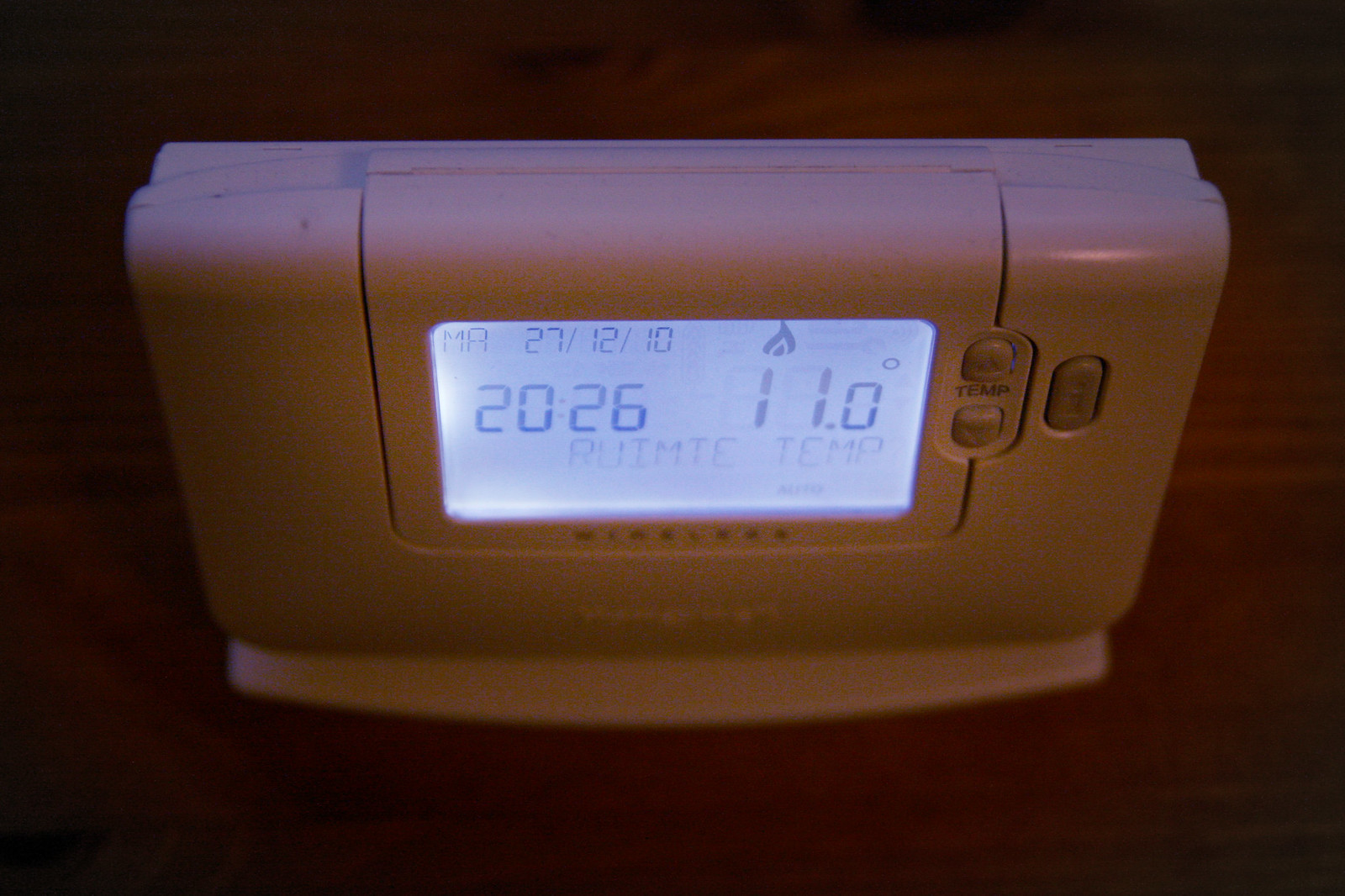The image depicts a white-cased thermostat mounted against a background that appears to be made of brown, wood-like material. The thermostat features a rectangular screen with curved corners, which is illuminated. On the right side of the thermostat, there are two buttons labeled "TEMP" - an up arrow button positioned above a down arrow button - for adjusting the temperature.

The screen displays several pieces of information: the date, shown as 27/12/10, the current time, which is 20:26 (8:26 PM), and the current temperature reading, which is 11.0 degrees. Below the temperature reading, the screen shows the label "Realmech temperature."